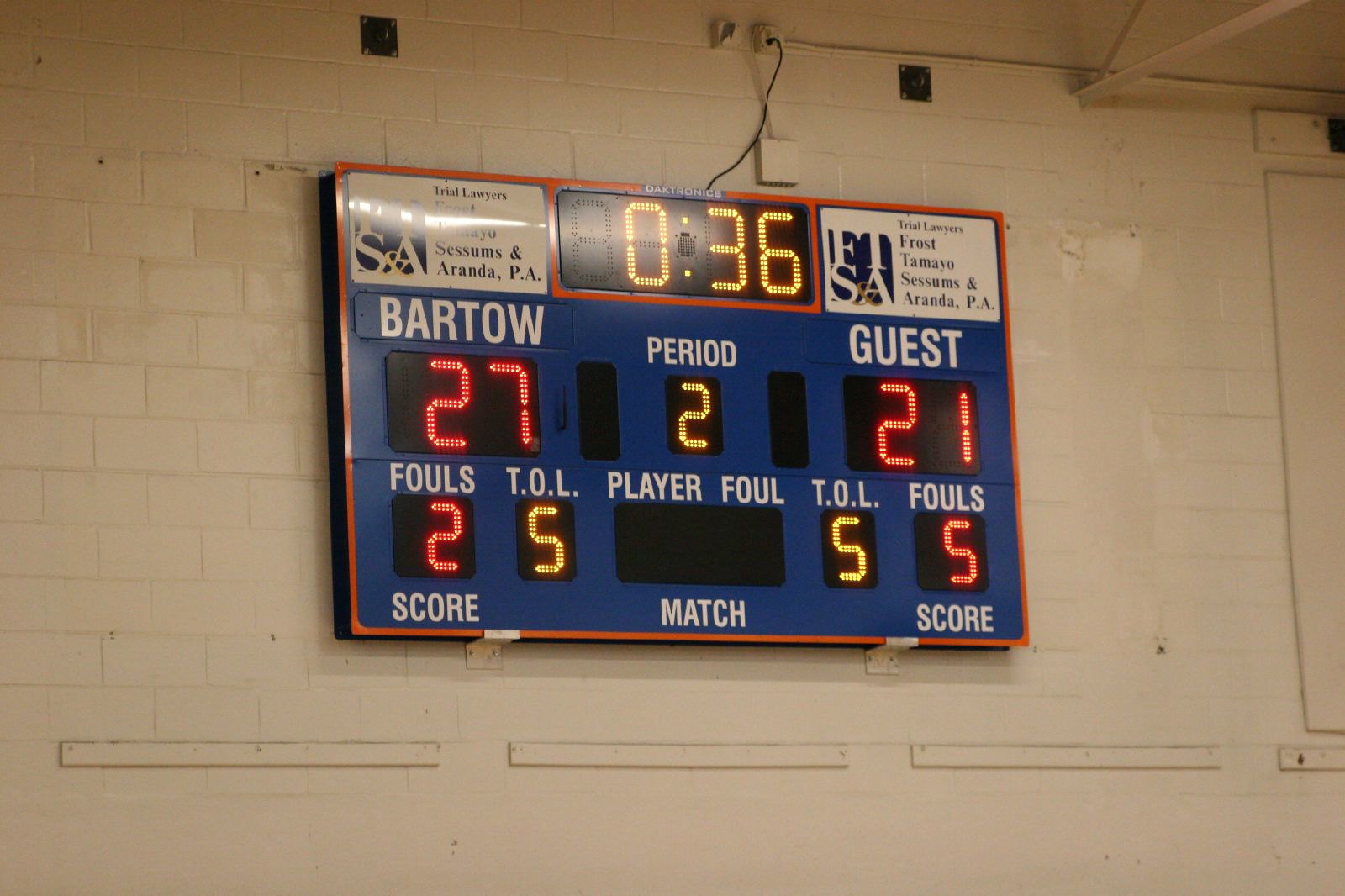This detailed photograph showcases a scoreboard prominently installed on a white-painted brick wall, likely located in a school gymnasium. The horizontally rectangular scoreboard is encased in a blue border with a thin orange outline. At the top center, a timer displays 0 minutes and 36 seconds in bold yellow block numbers. Flanking the timer on both sides are advertisements; both feature the same blue square and white rectangle design, with text reading "FTSA" and "Trial Lawyers: Frost, Tamayo, Sessoms, and Aranda, P.A."

On the scoreboard’s left side, "Bartow" is displayed in white letters with the current score of 27 in red electronic numerals beneath it. In the middle, "Period" is written in white with a yellow '2' below it, indicating the second period. To the right, "Guest" is labeled in white, and below it, the guest team’s score is shown as 21 in red numerals.

The bottom section of the scoreboard has several smaller sections for fouls, timeouts left (TOL), and player fouls. Bartow has accumulated two fouls and has five timeouts left, while the guest team has five fouls and also five timeouts remaining. The lower part of the scoreboard includes labels for "Score," "Match," and "Score" again in white lettering from left to right respectively.